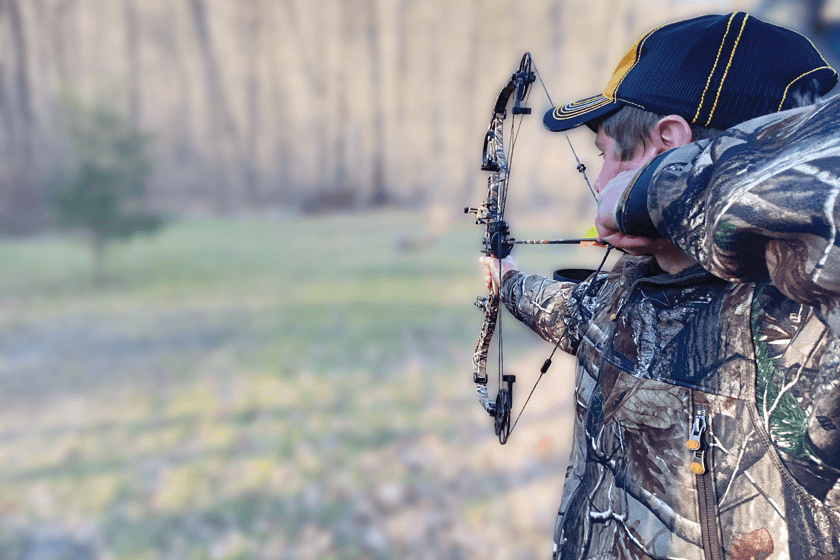The image is a color photograph in landscape orientation featuring a young man deeply focused on archery. He is captured in mid-action, standing on the right side of the frame while aiming at an indistinct target to the left. The man, who has short brown hair, is dressed in a camouflage jacket adorned in a pattern of leaves, twigs, and sticks in shades of brown, green, and beige. He wears a navy blue cap with distinctive orange stitching along the edges. The black compound bow is drawn back fully, with the arrow aligned and the quiver pressed close to his cheek, his eyes intently following the arrow's trajectory. His left hand pulls the bowstring back up to his ear, while his right side, including the elbow, is partially cropped out of the image. The bow features a yellow tail feather, indicating it is designed for hunting. The background is a blurred mix of green grass, a solitary tree to the image's left, and tall, barren trees further back, emphasizing the sharp focus on the archer's concentration and form. The overall style of this photograph is representational realism, capturing the precise moment with striking clarity and detail.